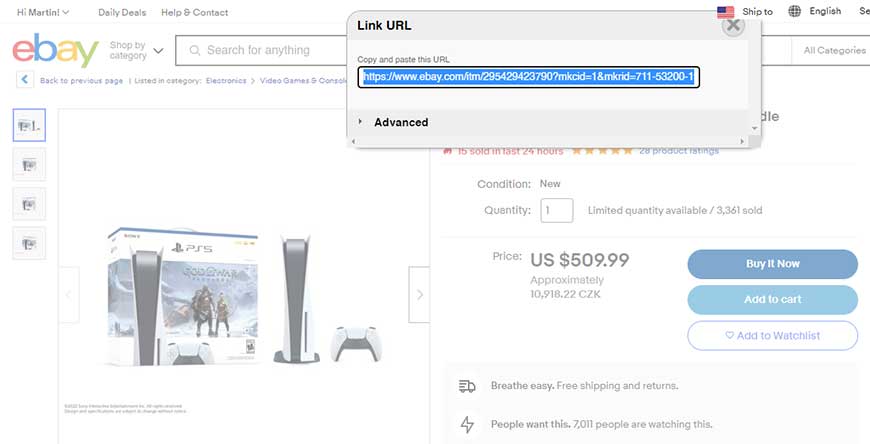The image features a white and grey color scheme with a URL link displayed within a rectangular box at its center. Beneath the rectangular box, there is smaller text instructing viewers to "copy and paste this URL." The URL within the field is already highlighted. Below the highlighted field, the word "Advanced" is prominently displayed in bold black text. In the top left corner of the rectangular box, the eBay logo is visible, with the letters "e" in red, "b" in blue, "a" in yellow, and "y" in green. The overall background of the image appears slightly blurry, focusing attention on the central details.